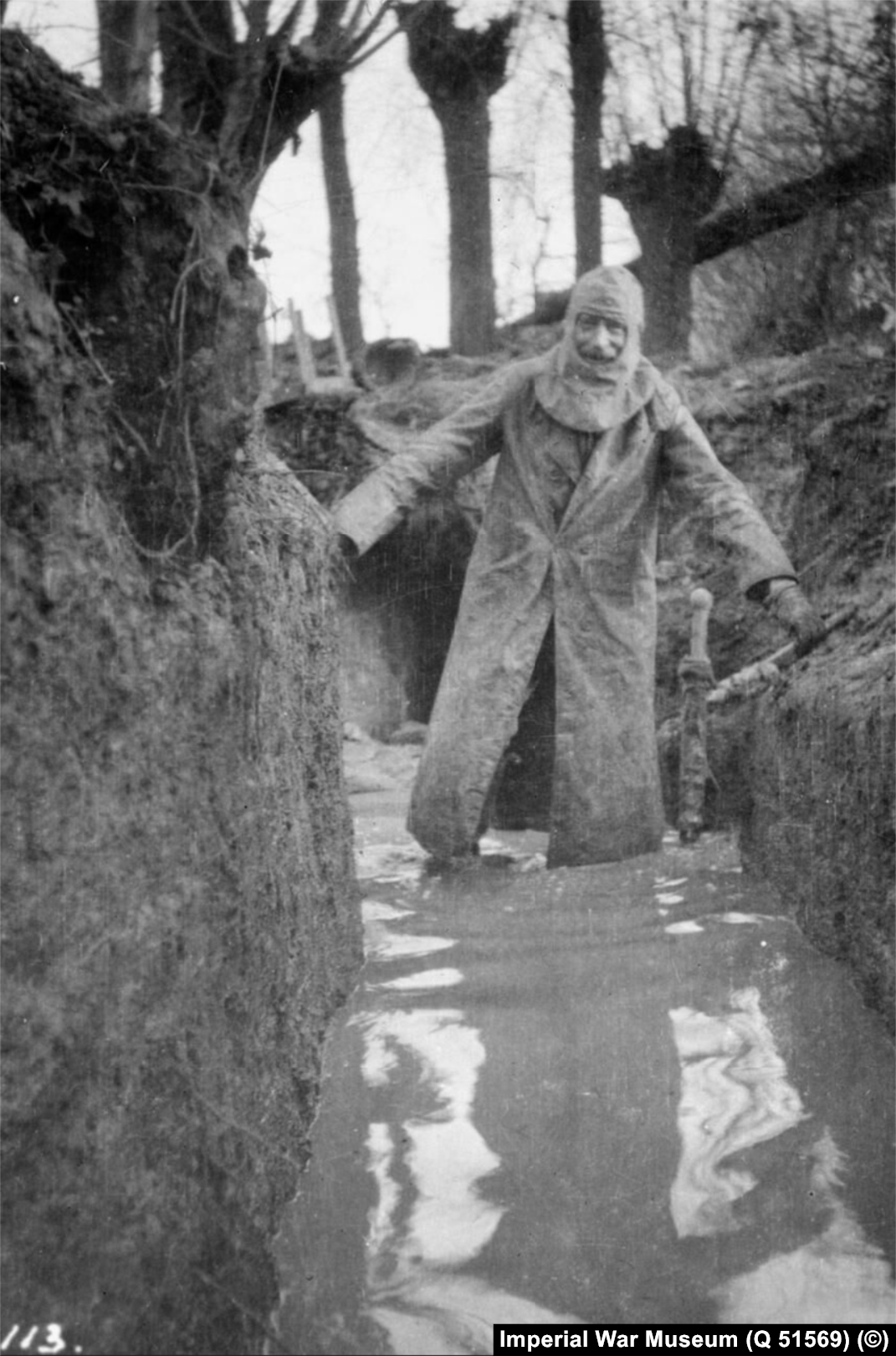This old, black-and-white photograph, labeled as 1 out of 3 with the inscription "Imperial War Museum Q51569," captures a man navigating a narrow, muddy trench. Portrayed in mid-tones of gray, black, and white, the photograph lacks sharp focus but vividly showcases the man’s shadow, which extends from the middle towards the bottom of the image. The trench's high, sod walls flank the man on either side, suggesting it could be a war-time shelter, often referred to as a dugout, used to protect soldiers from enemy fire.

The man, dressed in a long trench coat and some type of headgear, appears to be trudging through murky water or mud, possibly the aftermath of rainfall. His hands touch the walls for balance as he looks straight ahead, tolerating his harsh environment. The bare trees in the backdrop suggest a winter setting. A reflective surface beneath him hints that he is indeed wading through water, with the depth indicated by the disparity in wall heights around him. Despite the somber setting, this photograph, preserved by the Imperial War Museum, remains a poignant glimpse into the trenches of wartime, marked with the catalog number Q51569.